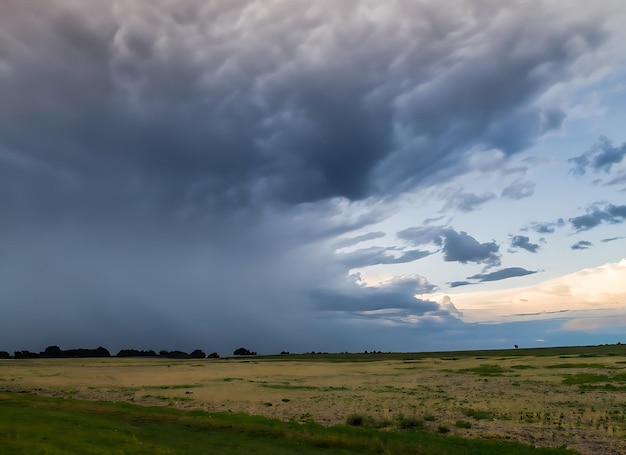This image captures a vast, open field under a dramatic sky, offering contrasting atmospheric conditions. The foreground of the image showcases healthy, short green grass, expanding into a patchier area with green interspersed among browner, yellower, and grayer patches suggestive of dead or bare earth. The horizon features a sparse line of trees concentrated to the left, becoming sparser towards the right, with some indistinct shapes that could be shrubs, bushes, or even a cow. Dominating the sky, the left side is marked by dark, stormy clouds, almost blending into a single mass indicative of an impending storm or tornado. In contrast, the right side transitions to a clearer sky with broken light clouds and a hint of blue sky, reflecting possible sunshine behind the clouds. This juxtaposition highlights the dynamic weather, with the stormy menace of the left giving way to a brighter, albeit still cloudy, expanse on the right.